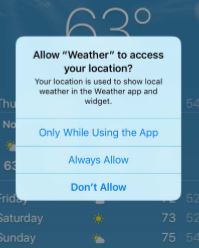A detailed screenshot of a weather application interface is partially obscured by a pop-up window. The visible portion of the app indicates a current temperature of 63 degrees Fahrenheit, with a forecast showing temperatures of 73 degrees for Saturday and 75 degrees for Sunday. The central focus of the image is a pop-up window requesting location access with the text: "Allow weather to access your location. Your location is used to show local weather in the weather app and widget." Below this message are three options: "Only while using the app," "Always allow," and "Don't allow." The image is strictly a digital interface display, with no photographic elements or presence of people, animals, birds, plants, trees, buildings, or any other real-world objects.